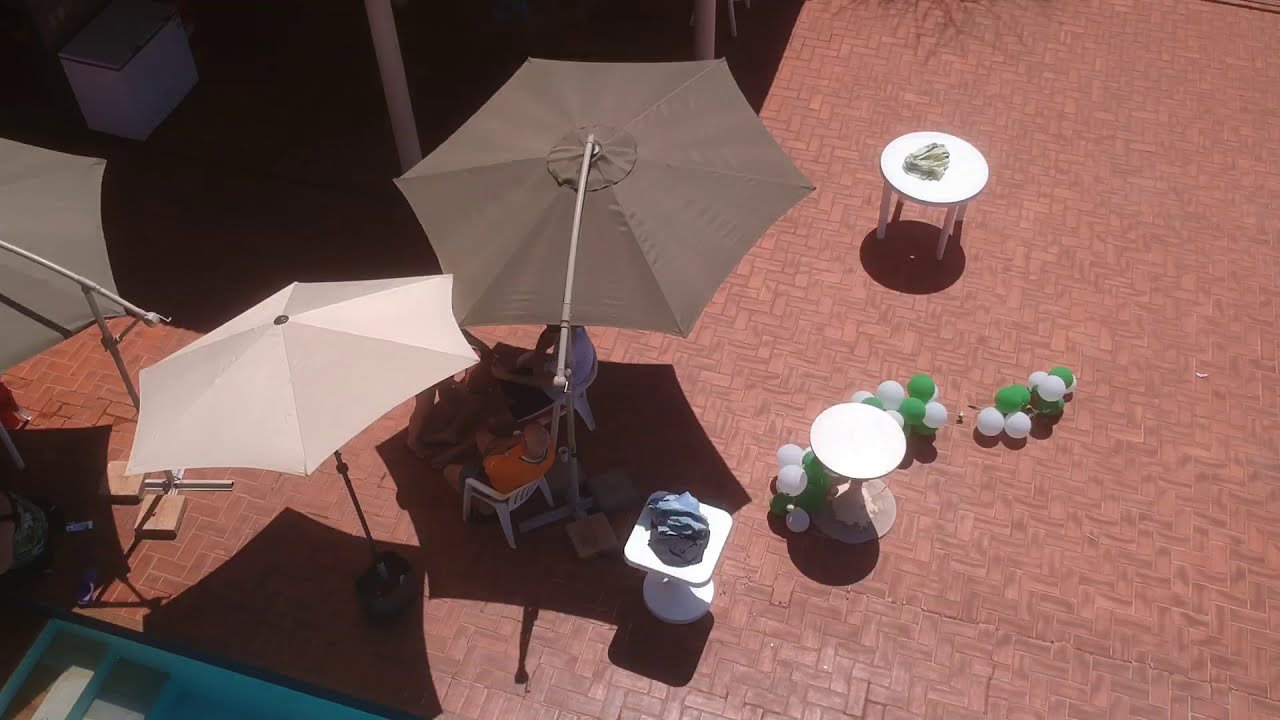The image depicts an outdoor patio scene, evidently taken in the middle of a sunny day. The ground is laid out with red brick flooring, flooded with bright sunlight. Central to the image are several people seated on white plastic chairs, comfortably positioned under a large, colorful beach umbrella, with another umbrella casting a shadow nearby. Among the seated individuals, one gentleman in an orange t-shirt and blue shorts stands out, alongside another person in a white sweatshirt and another in a blue t-shirt. Scattered around the patio are white and green balloons, remnants suggesting a recent celebration. The patio also features a couple of circular white tables and in the bottom left corner, steps leading to a swimming pool. The upper part of the image is dominated by another large shadow, possibly from a canopy or nearby building, providing additional shade to the lively, summery setting.